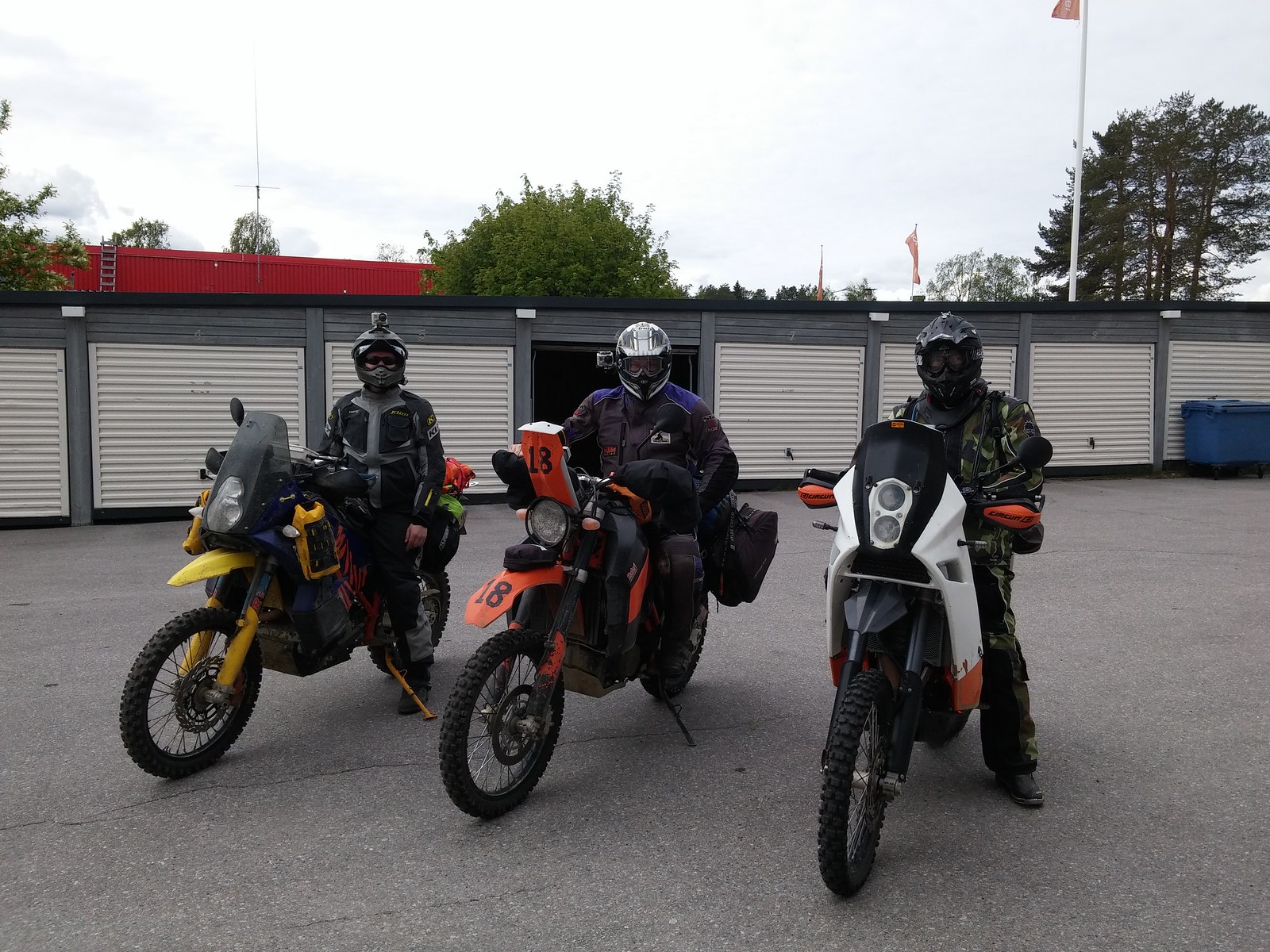This image captures three off-road-type motorbikes, each ridden by a fully-geared motorcyclist. The motorbikes are positioned in a row in front of an open storage unit, lending a sense of organization and readiness. On the left is a yellow motorbike, ridden by a person wearing a black helmet and protective gear, suggesting they are well-equipped for riding. In the middle, the orange motorbike prominently displays the number 18 in front of the wheel. Its rider contrasts with a blue jacket and white helmet, adding a splash of color to the scene. The rightmost motorbike is a mix of white and black with orange detailing, ridden by someone in a white jacket and green vest, topped with a black helmet. Behind this organized trio, the setting includes a red building, verdant trees, and a blue dumpster, which frames the scene and hints at a utilitarian, possibly communal space. Despite their full riding gear, likely male based on their stance and build, the riders exude an enigmatic presence, ready for an adventure.